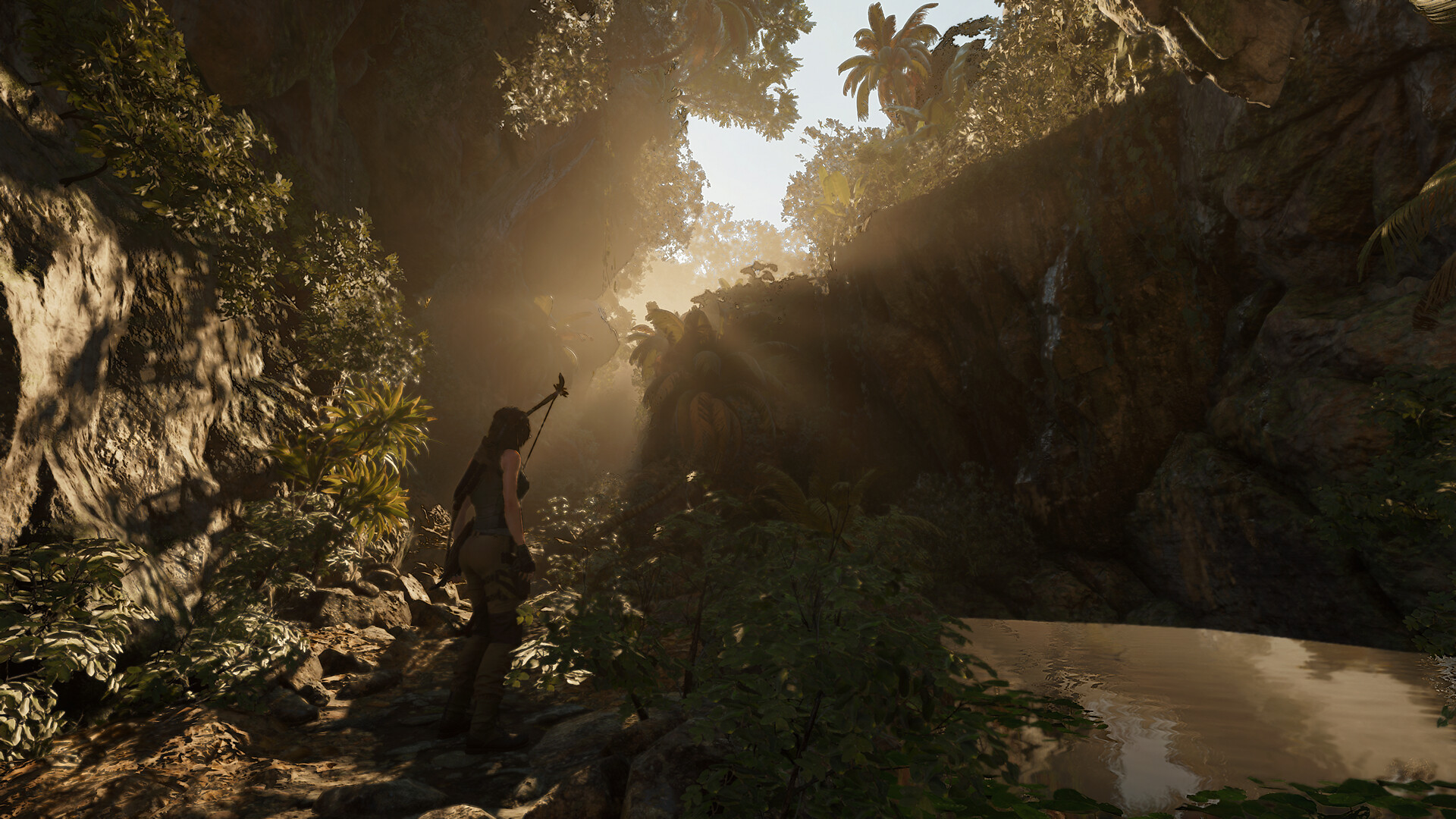The image appears to be a detailed screenshot from a video game, depicting a woman standing in a lush, dense jungle scene. She wears a green tank top and light green cargo pants, blending into the vibrant, natural surroundings. Over her shoulder, she carries a bow, and a quiver is slung on her back, suggesting she is equipped for adventure or combat. Her hands are clad in black gloves, and her brown hair cascades down as she stands on a pathway cutting through a canyon. The scene is backlit by sunlight peering over the cliff above, casting rays that partially illuminate her figure while leaving her partly in shadow, thanks to a rocky protuberance behind her. The environment around her is rich with tall jungle trees towering over the cliffs and a variety of bushes and shrubbery in both the foreground and background. In the lower right-hand corner, a body of water reflects the ambient light, adding to the immersive, verdant atmosphere of the scene.